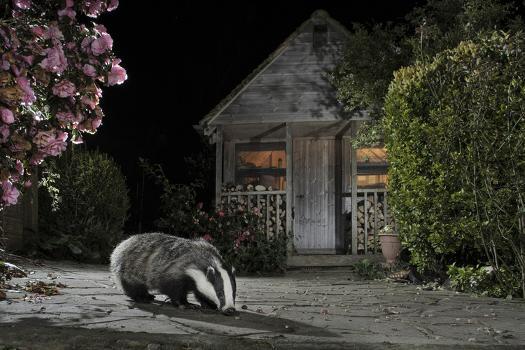This nighttime photograph, illuminated by an off-frame street lamp casting intense shadows, captures a gray badger with distinctive black and white face markings. The badger, its snout to the ground, is positioned on what appears to be a driveway or the front yard of a light gray-brown wooden cabin. The cabin, framed by greenery including a prominent pink rose bush hanging to the top left and another green bush to the right, features a small, partially obscured triangular-shaped front porch. The porch has stacks of wood behind its railings, and the house shows lights on in both windows flanking a central door, raised slightly off the ground. The sky is pitch black, emphasizing the nocturnal setting.